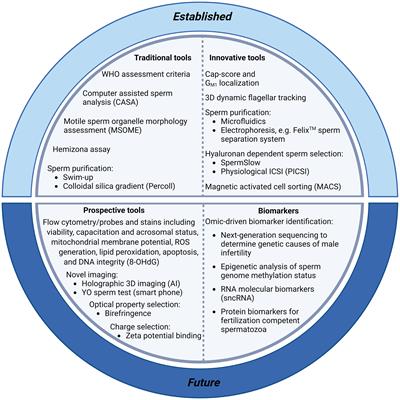The image features a circular diagram divided into four distinct sections, each labeled and containing various text elements. The outer barrier of the circle is two-toned: the top half is light blue and labeled "established" in small black text, while the bottom half is dark blue and labeled "future" in the same style of text.

The top-left quadrant of the circle is titled "Traditional Tools," with a series of black text listed beneath the heading. Adjacent to this, in the top-right quadrant, the section labeled "Innovative Tools" includes bulleted points and stylistic notes also in black text.

In the bottom half of the diagram, the bottom-left segment is labeled "Perspective Tools," featuring a paragraph followed by additional bullets and stylistic notes, all in black text. The bottom-right section is titled "Biomarkers," containing four bulleted points and stylistic notes of informational content.

The interior of the circle is white, featuring gray lining that separates each quadrant, giving the diagram a structured and organized appearance.